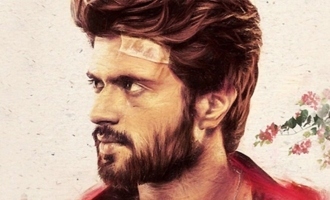The image features a striking profile shot of an Indian male with tan, caramel-colored skin, looking to his right. He has thick, wavy dark brown hair that reaches down to the back of his neck, partially covering his ears. His expressive brown eyes are turned to the right, with his right eye slightly obscured by his nose. He sports a full beard and mustache that frame his face and extend up to his hairline. A diagonal bandage is prominently placed on his forehead, just above his left eye, reaching up to his hairline. He is dressed in a red shirt, although only the top of his shoulders is visible in the small rectangular landscape image. The background is a light beige color, with a floor pattern and reddish-colored flowers with green leaves emerging from the right side, contributing to the drawn aesthetic of the image. He has a contemplative or intense expression, and the artist seems to have focused on the intricate details of his features and surroundings.